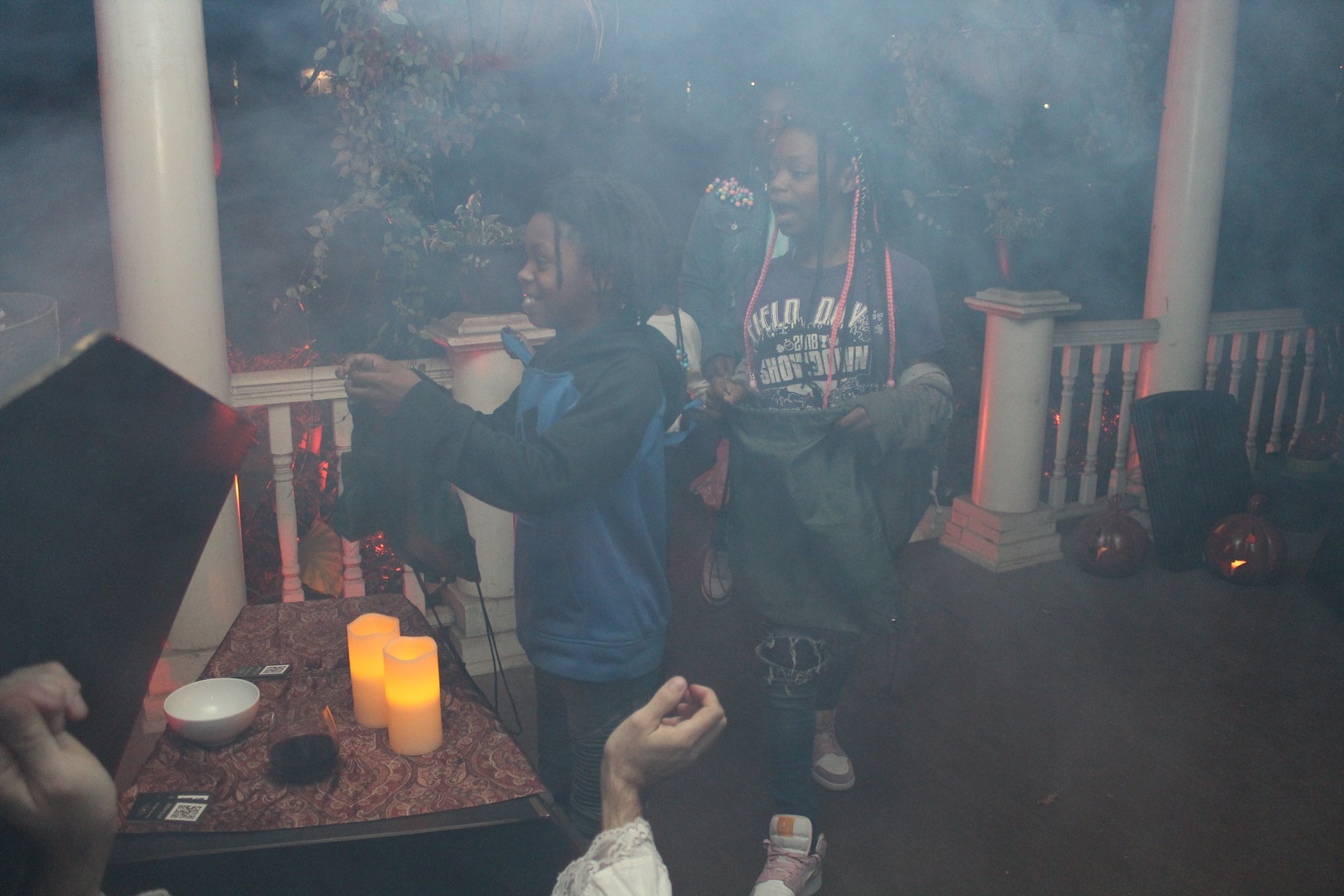The photograph, taken outdoors at night, captures a scene on a patio, likely someone's front or back porch, with the setting illuminated by candles scattered across a table. The image is slightly blurry, shrouded in a smoky haze which could be from grilling or the candles themselves. The patio has distinct white pillars on either side, with a fence and an exit leading to stairs in the background. The porch floor is brown, enhancing the rustic outdoor ambiance.

Three black children are the focal point of the image. One boy, smiling, stands beside the table, which is covered with a cloth and carries a white bowl, an ashtray, a glass with a dark drink, and several yellowish candles. He is dressed in a blue and black hooded sweatshirt and has long hair. Beside him stands a girl, slightly taller, who sports a blue t-shirt with white text and long hair adorned with brightly colored accessories, including pink accents. She wears pink sneakers. Behind her, partially obscured by the smoke, stands another girl.

The atmosphere of the porch includes additional details like a couple of pumpkins placed on the lower right-hand side, adding a touch of seasonal decoration. In the lower left-hand corner, a pair of older, Caucasian hands appears, reaching into the frame, adding to the sense of candid, rustic charm of the scene.